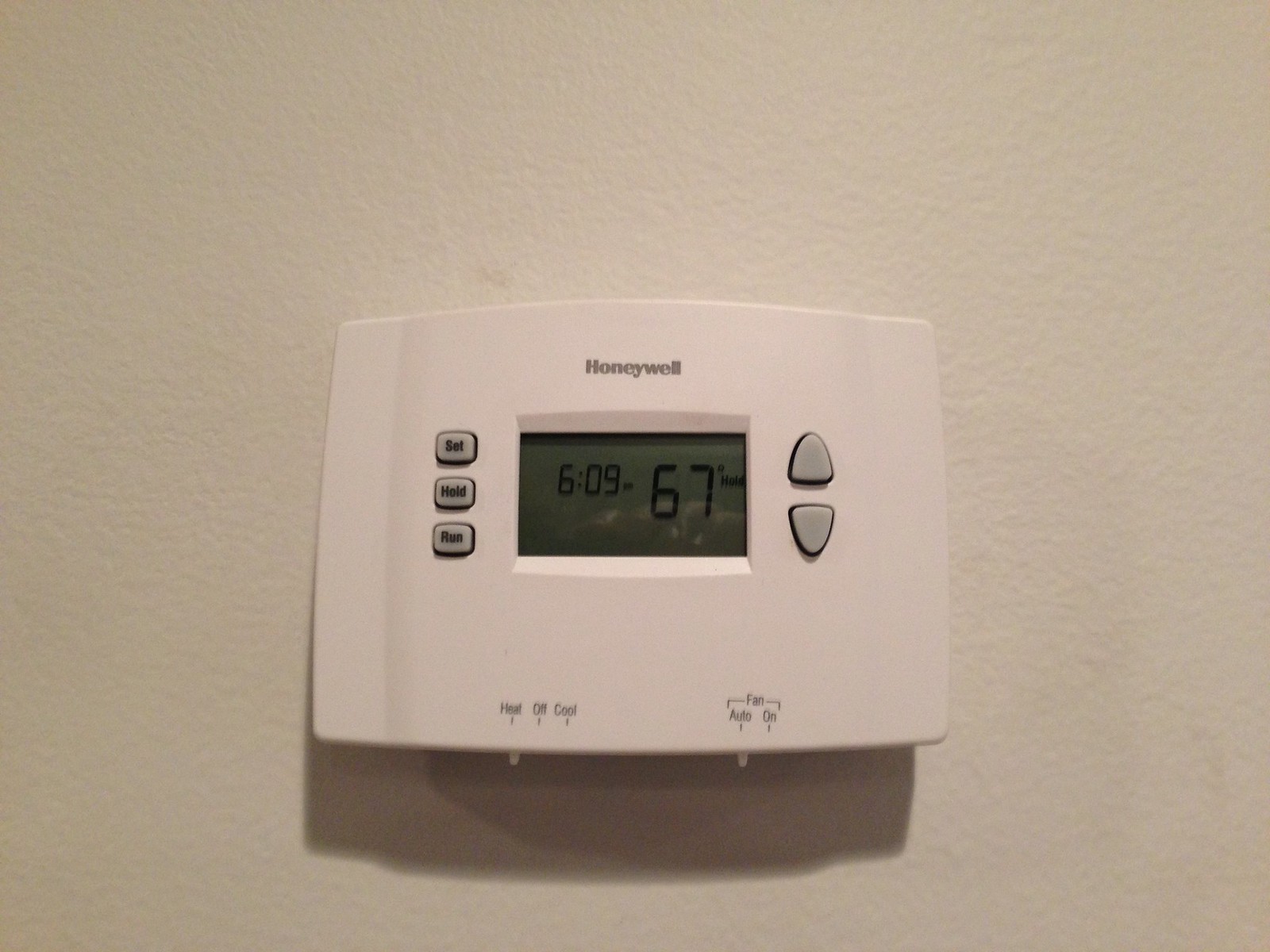The image features a Honeywell thermostat prominently centered against a plain cream-colored wall background. The thermostat itself matches the wall in a similar cream shade and has a short rectangular shape. At the top, the Honeywell brand name is clearly visible. Directly below the branding, the digital display shows the current temperature setting at 67°F and the time at 6:09 PM. Situated on the left side of the display are three buttons labeled "Set," "Hold," and "Run." To the right of the temperature reading are two buttons for adjusting the temperature up or down. The bottom section of the thermostat displays the system's mode controls, with "Heat," "Off," and "Cool" settings visibly marked; it is currently set to "Heat." Additionally, to the right of these controls are the fan settings "Auto" and "On," with the fan set to "Auto."